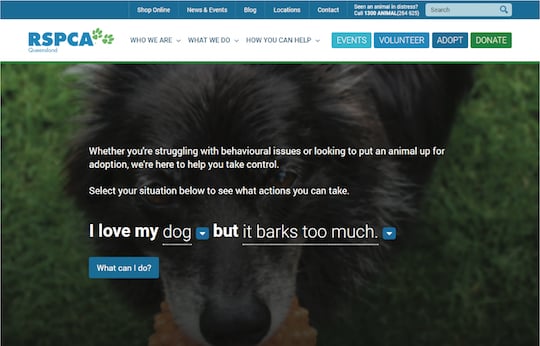This image depicts the homepage of the R.S.P.C.A. online store, featuring a well-organized and user-friendly interface. The store's name, "R.S.P.C.A.," is prominently displayed in blue. The navigation bar includes drop-down menus titled "Who Are We," "What We Do," "How You Can Help," and "Events," each providing quick access to various information and resources. Additional options like "Volunteer," "Adopt," and "Donate" are highlighted in blue and green.

At the top, users can find links to "Shop," "Online," "News and Events," "Blog," "Location," and "Contact," alongside a search bar for easy navigation. Centrally featured is a striking image of a black and white dog playfully biting a yellow toy, set against a lush green grass background.

Below the image, there is a descriptive text: "Whether you are struggling with behavioral issues or looking to put an animal up for adoption, we are here to help you take control. Select your situation below to see what actions you can take." This message is followed by a sentence with two interactive drop-down menus, "I love my dog, but it barks too much," allowing users to explore specific details related to their situation.

A prominent blue button labeled "What Can I Do?" in white text encourages users to seek assistance. Clicking the first drop-down menu, placed after "I love my dog," provides details about expressing affection for a dog. The second drop-down, following "but it barks too much," offers guidance on managing excessive barking. This thoughtful design enables users to address their concerns and find solutions effectively.